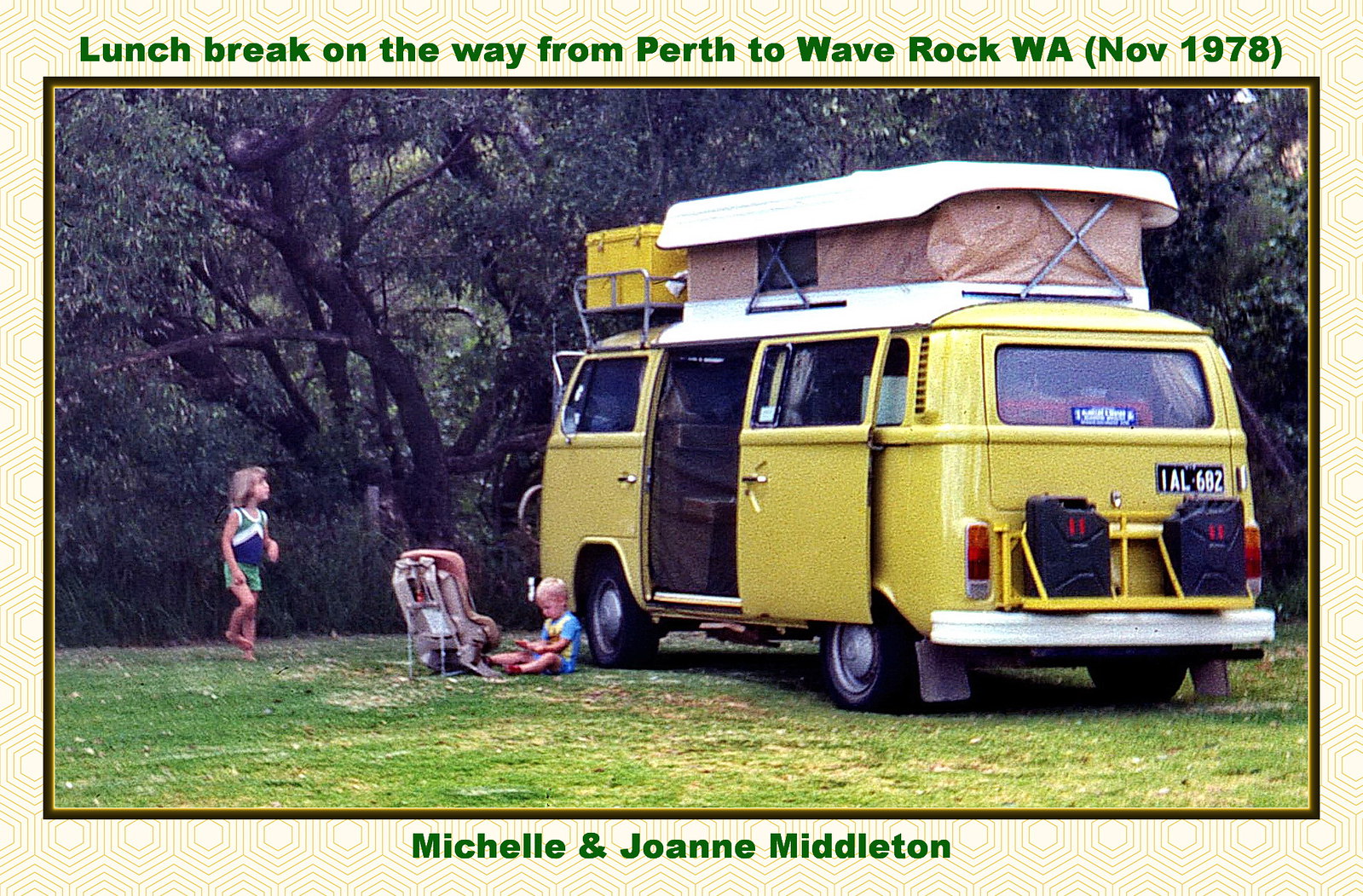An old yellow Volkswagen van, with its sliding door wide open and the pop-top extended upwards, sits prominently in the center. The roof is a contrasting white with a light brown lining and is supported by silver X-braces. Attached to the back, a brace holds several black gas cans adorned with red numbers. Blue rubber stickers with white text decorate the back window. A black license plate with white letters reads "IAL 682."

To the left of the van, two children are visible: one stands facing the van, wearing green shorts and a colorful shirt featuring blue at the top, a white stripe in the middle, gray-green sections, and white circles. Near the front wheel of the van, another child sits with hands outstretched, wearing a yellow and white shirt. In front of this seated child is a child safety seat.

Encircling the entire image is a border adorned with intricate diamond patterns. At the top of the border is green text that reads "Lunch break on the way from Perth to Wave Rock, WA, November 1978." Along the bottom of the border, the names "Michelle and Joanne Middleton" are inscribed.